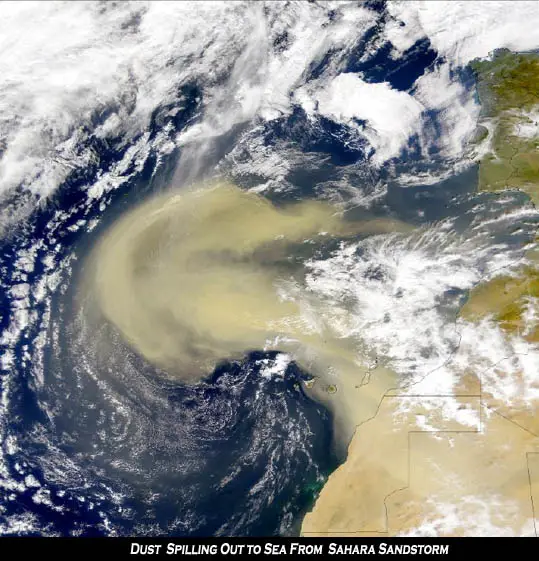This is a detailed satellite image capturing a significant sandstorm originating from the Sahara Desert in Africa. At the bottom of the image, a caption reads "Dust spilling out to sea from Sahara sandstorm." The image prominently displays a vast brown cloud of dust spreading into the blue ocean waters, indicating the extensive reach of the sandstorm. White swirls of turbulent clouds are also visible, surrounding the center of the dust storm, suggesting where the eye of the storm might be. Additionally, parts of the African landmass border, with distinct land formations, are discernible in the lower right corner of the photograph. The overall hues in the image range from white and gray clouds to a striking blue ocean and light brown dust, giving a vivid depiction of this natural event.